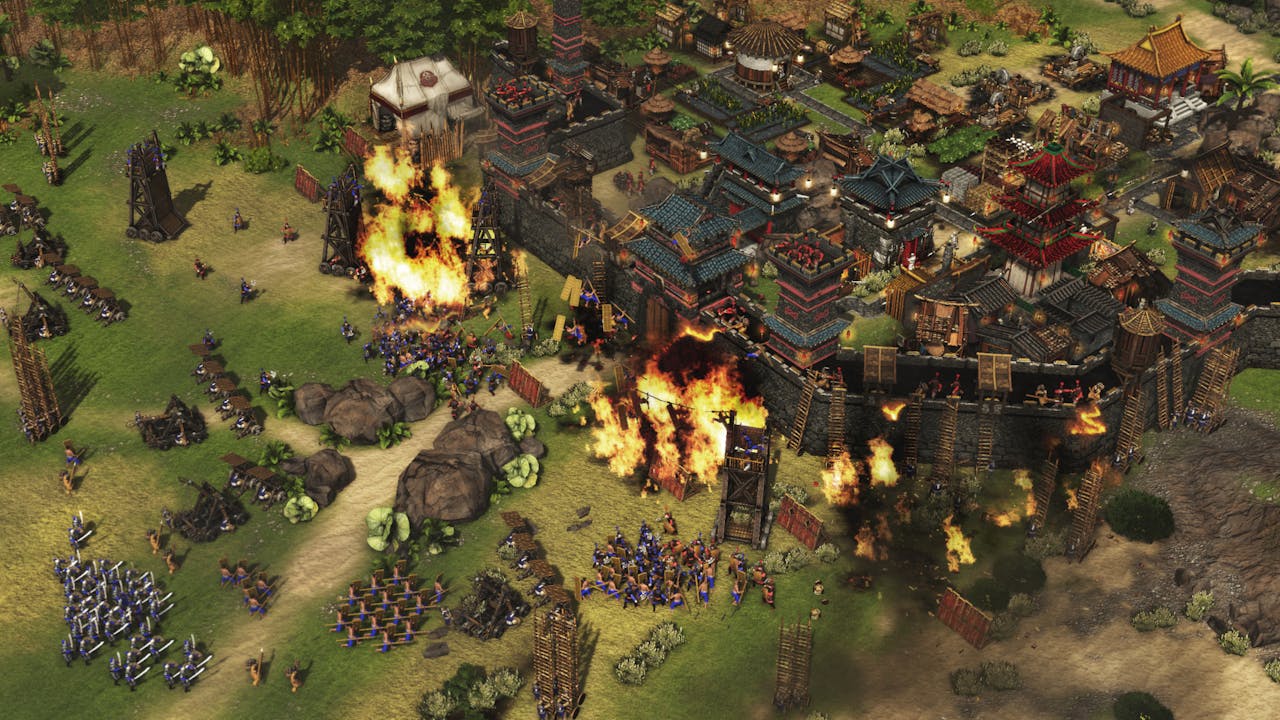The image portrays a vivid, action-packed scene from a photorealistic computer game set in what appears to be medieval Japan. The foreground features a large wooden fortress or a fortified town on the right, under siege by numerous small attacking forces from the left. The perspective is a bird's eye view, revealing detailed but non-specific outlines of grouped soldiers advancing towards the fortress.

Six to seven towering wooden siege engines dominate the landscape, with several large red-orange fires blazing amongst them. The attacking army is clearly determined, with soldiers wielding spears and makeshift shields, and some attempting to scale the fortress walls. Visible behind these walls are Asian-style structures, further indicating a culturally rich, digitally crafted setting.

The fortress itself is also ablaze in multiple locations, adding to the chaotic atmosphere. Despite the vivid colors, particularly the greens and browns of the landscape, the primary visual focus is the dramatic spread of fire and the intense struggle between the defenders and the invaders, encapsulating the game's dynamic and immersive warfare experience.